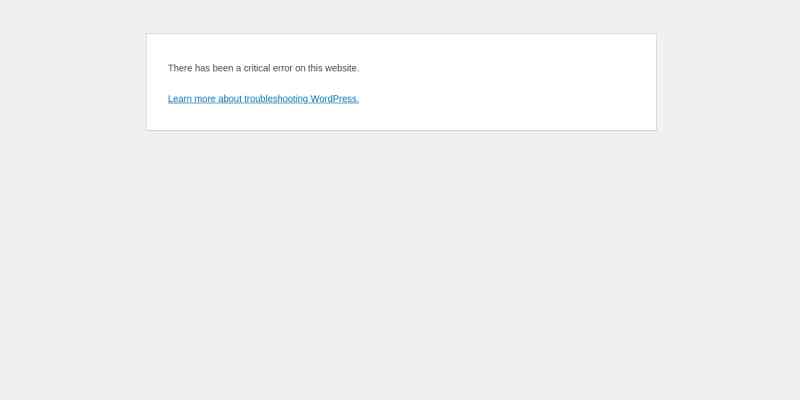This is a detailed screenshot capturing an error message from a WordPress website. The image appears to be square or rectangular in shape with a predominantly white background. Positioned in the upper left corner, there is a small text written in medium gray that states, "There has been a critical error on this website." Directly below this message, in a bright blue, underlined font, is a hyperlink reading, "Learn more about troubleshooting dot wordpress." This link likely directs users to a resource for addressing and resolving the error. The text is presented in a standard, legible font. The overall composition of the screenshot is minimalist, highlighting the critical error message and providing a clear pathway for obtaining more information through the provided link.